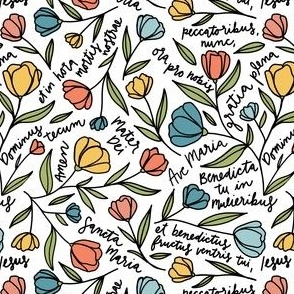The image features a simple yet vibrant hand-drawn art of various types of flowers set against a white backdrop. The flowers, approximately 20 in number, come in a variety of colors including yellows, blues, reds, pinks, and teals, each uniquely shaded. Each flower comprises three petals at the forefront with a few smaller petals behind and is positioned randomly but gracefully, facing different directions—some pointing upwards, while others face left, right, or down.

Among the stylized flora, thin black lines form the stems, occasionally accented with small leaves. Scattered throughout the image are cursive black texts, including names and phrases like "Ave Maria," "Samantha Maria," "Benedicta," and "Amen," inscribed between the floral arrangements. The overall composition is visually appealing, digitally rendered to enhance the bright and diverse colors of the flowers, evoking a lively and cheerful atmosphere.